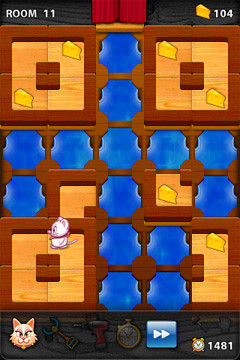**Caption**: This nostalgic image showcases an early vintage video game screen, reflecting the simplicity and charm of gaming's formative years. The layout is straightforward, featuring a mix of blue vertical and horizontal pieces arranged in the center, creating pathways for the characters. A small, smiling mouse character traverses the screen, seemingly in pursuit of slices of cheese scattered throughout the game. 

The lower left corner displays a sneaky-looking cat, poised to threaten the unsuspecting mouse should it wander too close. The game screen is speckled with brown and tan areas, adding a rustic touch to the overall aesthetic. Players navigate through the game by moving blue pieces and cheese slices vertically and horizontally.

In the game's interface, the upper left corner is labeled "Room 11," while the upper right corner shows a cheese icon with the number "104" beside it, likely indicating the amount of cheese collected or available. The lower right corner features an alarm clock icon with the number "1481," possibly representing a countdown or score. The mouse and the cat are separated by several squares, with the mouse positioned at a safe distance from its feline adversary, further adding to the strategic depth of the game.